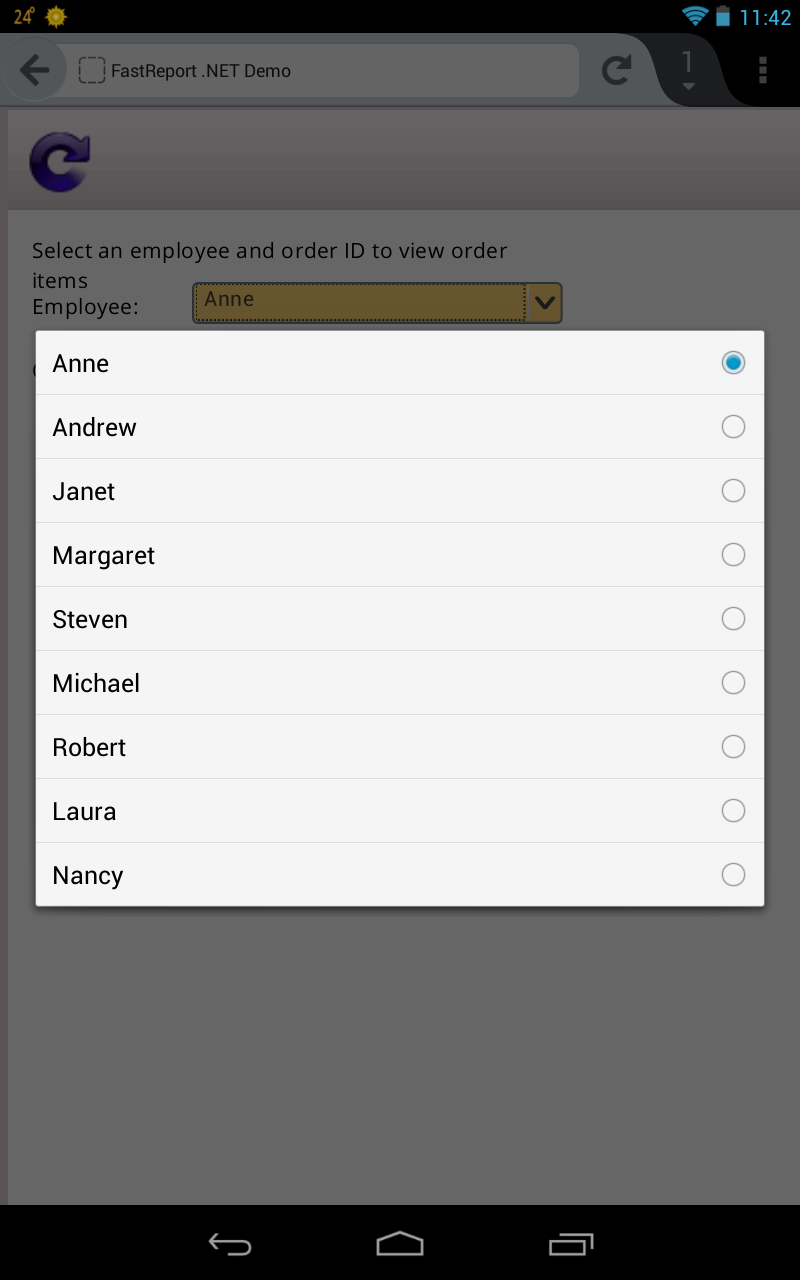The image depicts a digital interface, most likely a mobile device screen with a temperature reading and an employee selection tool. At the top, there is a solid black bar. Below it, in bold blue text, it reads "24" next to a sun icon, indicating a temperature of 24°C. On the top right, there are blue icons for Wi-Fi signal strength and battery status, which appears almost full at 11:42 AM.

Underneath the status bar, there is a grayed-out left-facing arrow and a white search bar labeled "fastreport.datnemo." Next to the search bar are a refresh icon, a number "1," and a menu indicated by three vertical dots. Below this, on a gray background, is another refresh button in blue.

The main content area, set on a white background with black text, features an interface where users can select an employee and order ID to view order items. The interface displays a list of employee names on the left side column and selection bubbles on the right. The first bubble, labeled "Anne," is selected and highlighted in blue. Below Anne, the names listed are Andrew, Janet, Margaret, Stephen, Michael, Robert, Laura, and Nancy.

At the bottom of the screen, there is another black bar including navigational icons left of center: a back arrow, a home button, and two overlapping squares indicating a task view or recent apps function. This image represents a clean and efficient employee management or selection tool interface, awaiting user input or action.